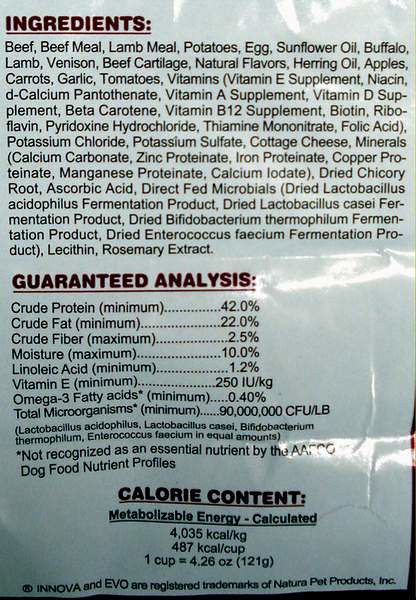This image shows the back of a white packet of pet food in portrait orientation, with the packet occupying nearly the entire frame save for a sliver of background on the right. At the top, the word "INGREDIENTS" is prominently displayed in bold, capitalized letters, colored in a brownish-red hue and underlined. Below this heading, a detailed list of ingredients appears in black text, each item starting with a capital letter. Key ingredients include beef, beef meal, lamb meal, potatoes, eggs, sunflower oil, buffalo, lamb, venison, and beef cartilage.

Midway down the packet, another section in red capital letters, underlined, reads "GUARANTEED ANALYSIS." This section enumerates the nutritional breakdown of the food, listing components such as crude protein, crude fat, crude fiber, moisture, linoleic acid, vitamin E, omega-3 fatty acids, and total microorganisms with their respective percentages. It includes a disclaimer stating that "extracts not recognized as an essential nutrient by the AAFFC dog food nutrient profiles."

At the bottom, the calorie content is detailed, providing both kilojoules and kilocalories, along with a measurement conversion indicating that one cup equals 4.26 ounces. The packet also identifies its manufacturers, Innova and Evo, which are registered trademarks of Natura Pet Products. The packaging material appears to be a crinkly type, possibly cardboard or plastic, adding to the textured look seen in the photo.